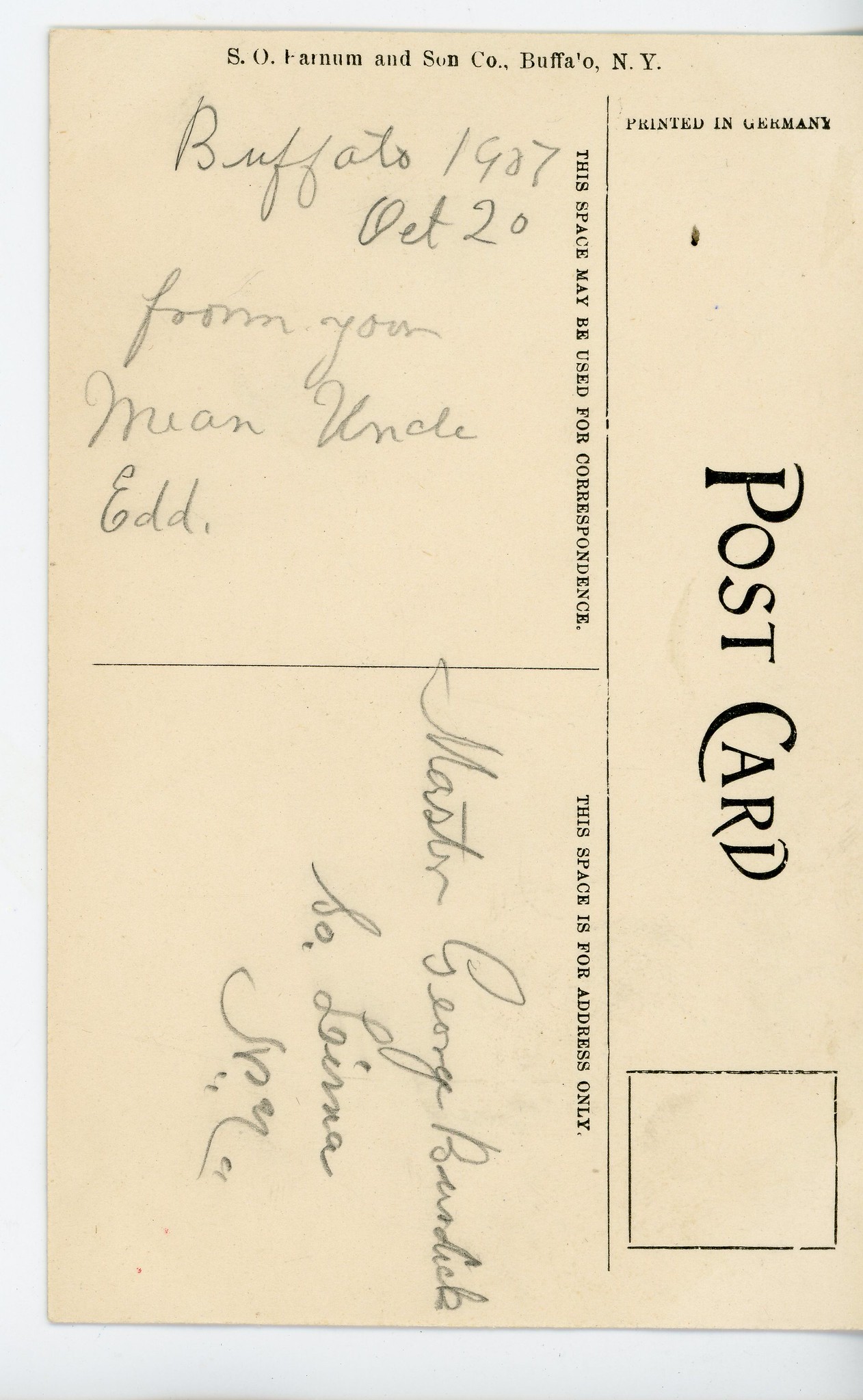A well-preserved postcard from Buffalo, dated October 20, 1907, is laid out on a white backdrop. This aged postcard, once presumably white, now appears yellowed or tan. The postcard is oriented vertically, and the front side is not visible. However, the back features distinctive details: at the top, in a black Art Deco-style font, it says "postcard" and includes a boxed area intended for a stamp, although no stamp is present. 

In cursive handwriting on the left-hand side, it reads, "Buffalo, 1907, October 20th, from your mean Uncle Ed," though one person noted it as "Eddie." Another section, designated for the address, contains the text "Master George Berndijk" (the last name being somewhat illegible and ending with either "k" or "dijck"), and “A.D. Loma” along with some Arabic characters that are not readable. The postcard also notes "printed in Germany" and contains, down one side, "Esso, Farnham and Sunco, Buffalo, New York." The cursive ink is black, contrasting against the postcard’s aged tan background.